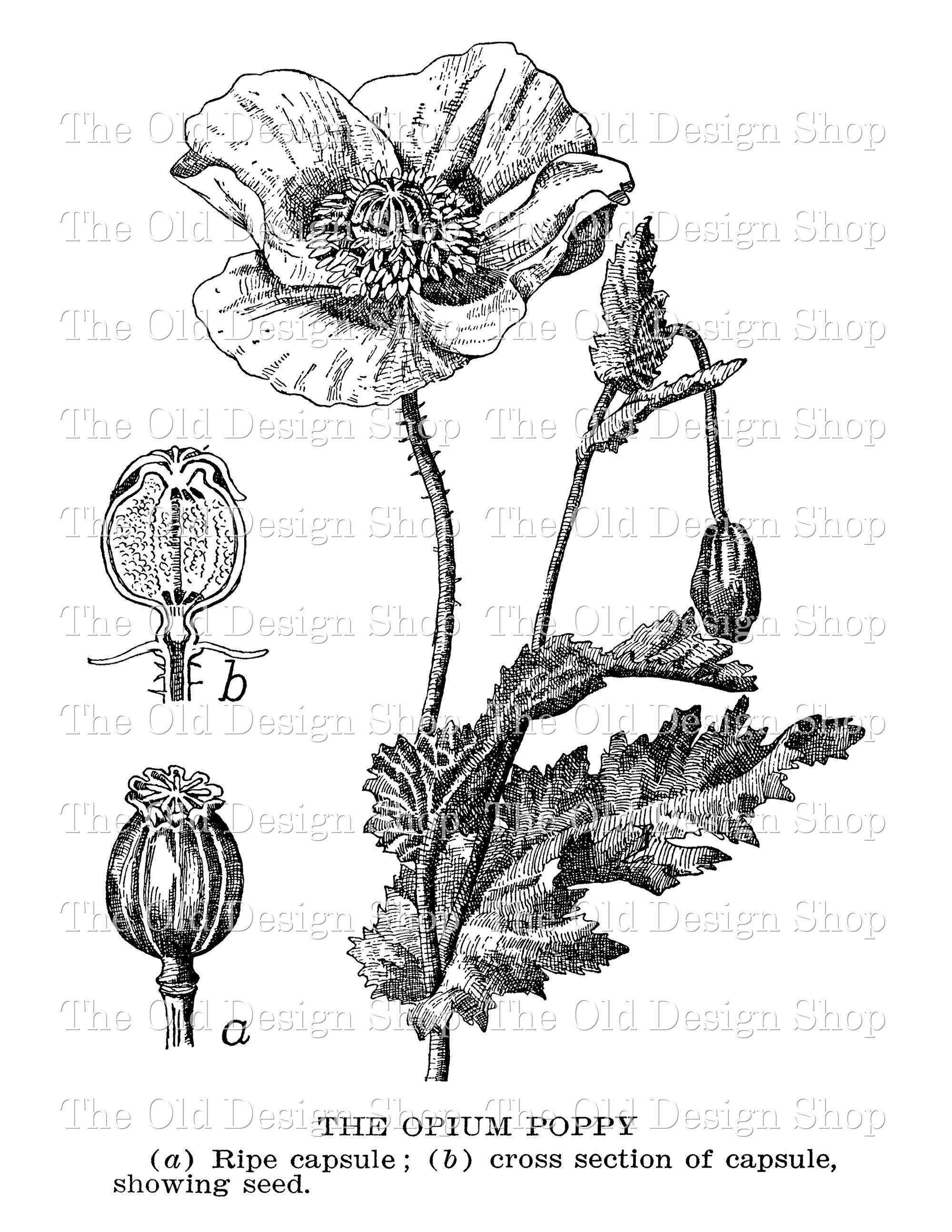This detailed scientific illustration, rendered in black and white pen and ink, captures the opium poppy with a precision reminiscent of 19th-century botanical drawings. The main image showcases a meticulously detailed poppy featuring a long, leafless stem ending in a bloom with prominent petals. At the base, the stem has one long and one smaller leaf. To the right, another stem carries a drooping bud and a stamen, adding depth to the composition. The left side of the illustration highlights two sub-illustrations: 'A' depicts a ripe capsule, and 'B' offers a cross-section showing the seeds inside. Below, uppercase text identifies the subject as "The Opium Poppy," with annotations for the sub-illustrations. The image is overlaid with a faint repeating watermark that reads "The Old Design Shop," giving it an archival feel. This detailed, photorealistic illustration exudes the fine craftsmanship and scientific accuracy typical of historical botanical art.